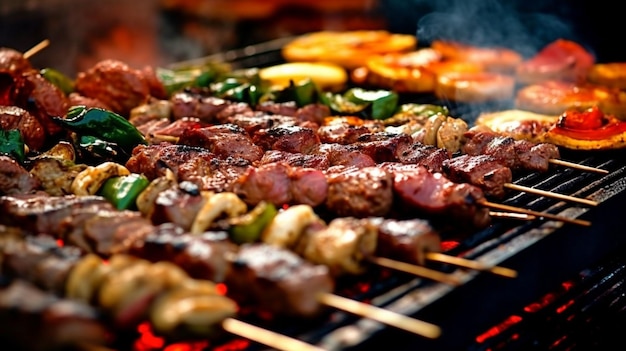This image captures a close-up, high-definition view of a fiery barbecue grill laden with a variety of skewered foods. The black iron surface of the grill is covered with around ten kebabs, each displaying a vibrant assortment of meats, vegetables, and even fruits. The kebabs feature different combinations, including chicken, pork, beef, shrimp, and various vegetables like green bell peppers, mushrooms, and potentially spinach or leafy greens. Some skewers appear to include colorful slices of orange and grapefruit. The glowing red coals beneath and the visible smoke rising from the grill emphasize the intense heat, while the vibrant colors of red, yellow, green, and cream showcase the freshness and diversity of the ingredients. The background is blurred, keeping the main focus on the skewers, which are slightly charred and emitting smoke and steam, indicating that they are being cooked to perfection.